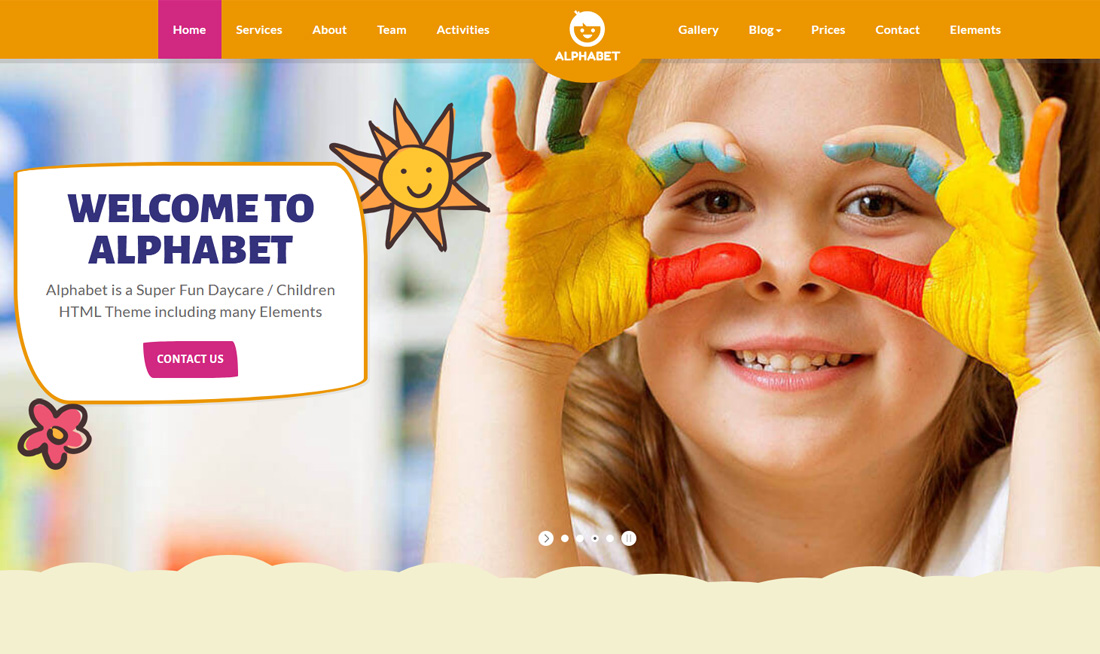Welcome to Alphabet! The homepage of the Alphabet website features a vibrant image of a joyful kindergarten girl with paint-covered hands. The palms of her hands are smeared with bright yellow paint, while each of her fingers displays a different color: red, blue, yellow, green, and orange. She has her hands playfully positioned around her eyes, mimicking a pair of eyeglasses, and is beaming with a big, cheerful smile. The site menu includes tabs for Home, Services, About, Team, Activities, Gallery, Blog, Prices, Contact, and Elements, all of which promise a super fun daycare experience for children.